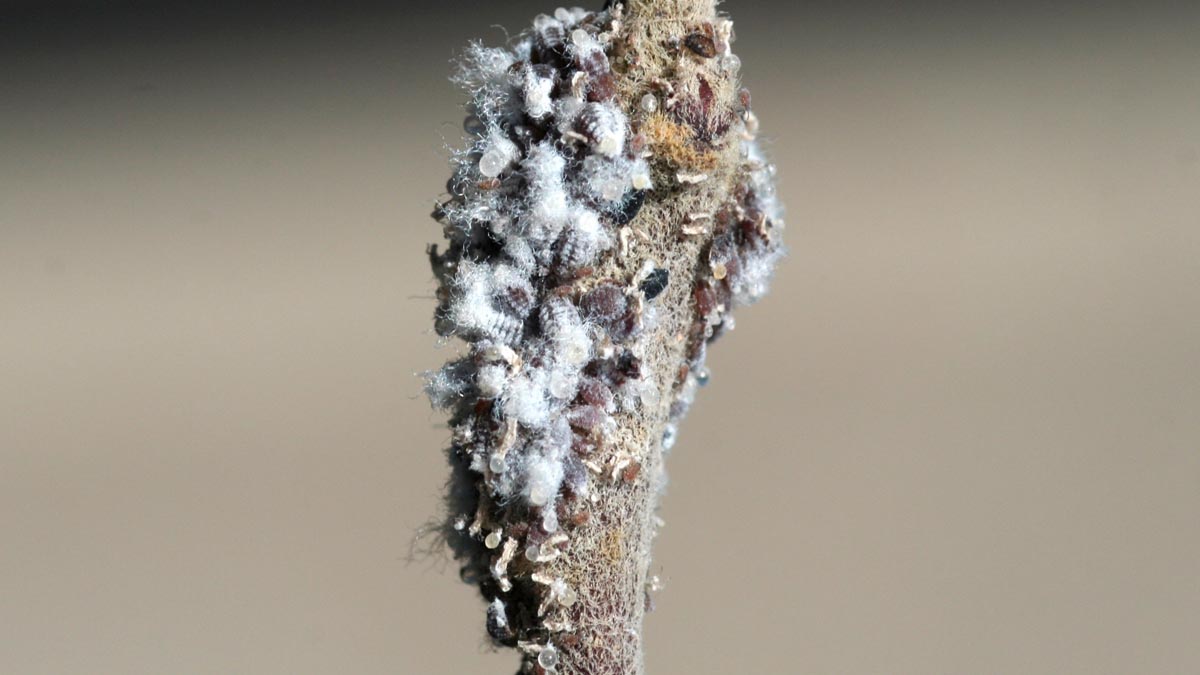The photograph appears to be a close-up, possibly taken in a natural outdoor setting. The background features a light brown, faded hue, suggesting a nature-like environment. Central to the image is a brown, brush-like tool or stick that emerges prominently from the lower middle. This stick is covered in numerous small objects that resemble insects, carrying a fluffy, sponge-like or white fuzzy substance. The minute details and the unclear nature of the items on the stick suggest it could be a microscopic image, capturing a scene where dust particles or tiny insects are perhaps trapped in the brush's fibers.